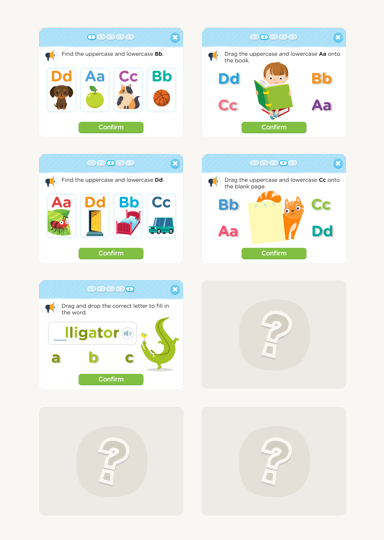A screenshot of a colorful and engaging language learning app designed for children features eight interactive sections, five of which are highlighted. The first section prompts users to find the uppercase and lowercase 'b' and 'B' among a row of letters (d, d, a, a, c, c, b, b), with a confirm button below to submit their choice. Upon pressing the correct button, it likely provides feedback such as "Yay, you did it!" or "Try again."

The second section depicts a child reading a book and instructs users to drag the uppercase and lowercase 'a' and 'A' onto the book from a selection of letters (a, a, b, b, c, c, d, d). The third section asks users to find the uppercase and lowercase 'd' and 'D' from another set of letters (a, a, d, d, b, b, c, c). 

In the fourth section, users are tasked with dragging the uppercase and lowercase 'c' and 'C' onto a blank page, with letter choices of (b, b, a, a, c, c, d, d).

Finally, the last active section challenges users to complete the word "alligator" by dragging and dropping the correct first letter from the options 'a,' 'b,' or 'c,' and to then click confirm.